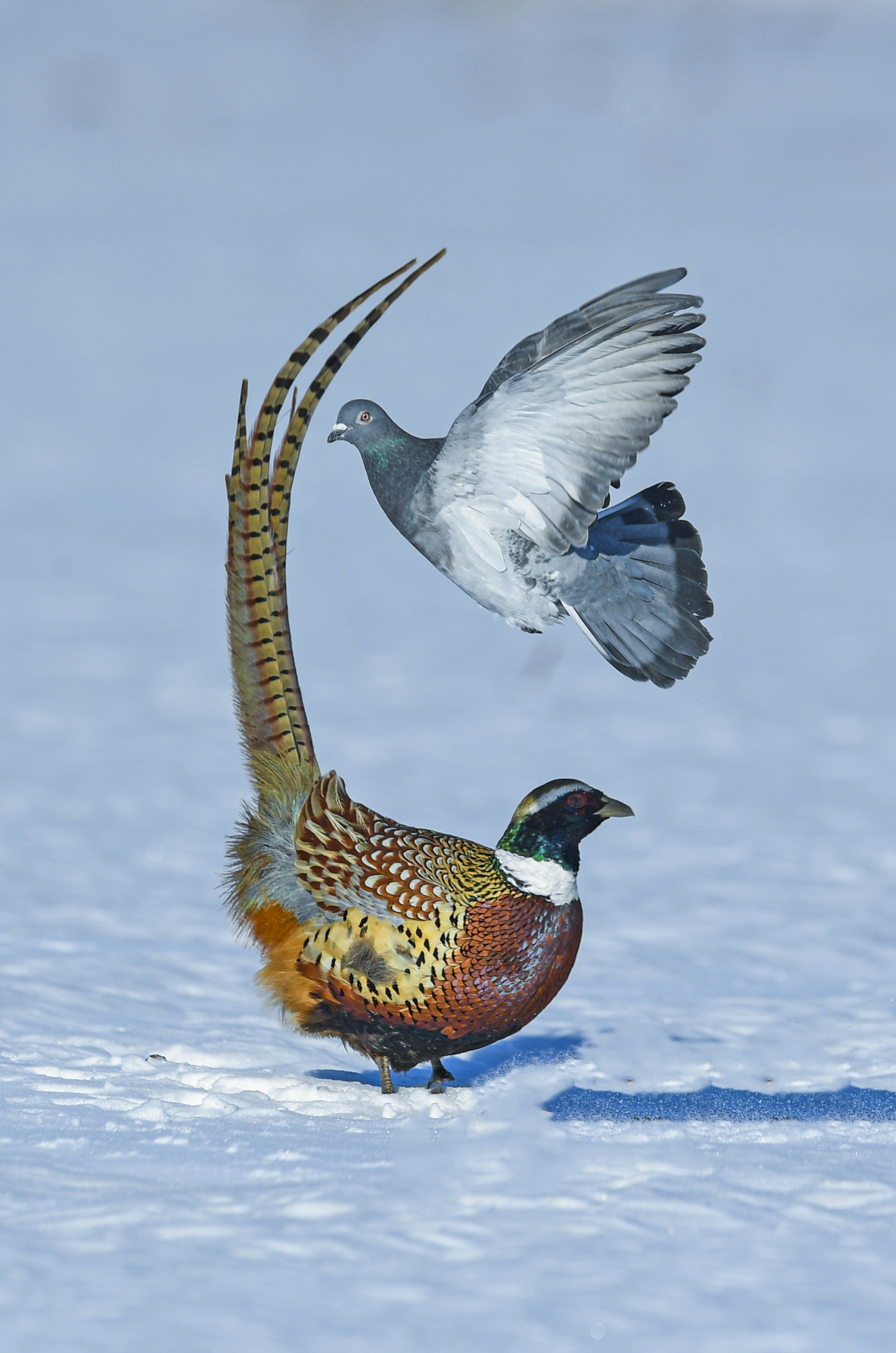In a stunning high-definition photograph likely captured by a wildlife photographer, two birds are vividly presented against a snow-covered, bluish-white outdoor background illuminated by sunlight. Centered in the image, a gray and white pigeon gracefully flies above a striking ring-necked pheasant, its wings widespread in motion. The pheasant, standing on the pristine white snow, boasts a vibrant appearance with a dark, possibly black or deep blue head transitioning into a distinct white ring around its neck. Its body exhibits a rich brown hue adorned with spotted patterns, while its long, arched tail features striking yellow and brown stripes. The pheasant's feet, a contrasting black, firmly rest on the snow, casting a clear shadow beside it, as does the pigeon mid-flight. This composition not only highlights the intricate details and colors of each bird but also captures the serene and chilly ambiance of their natural habitat.